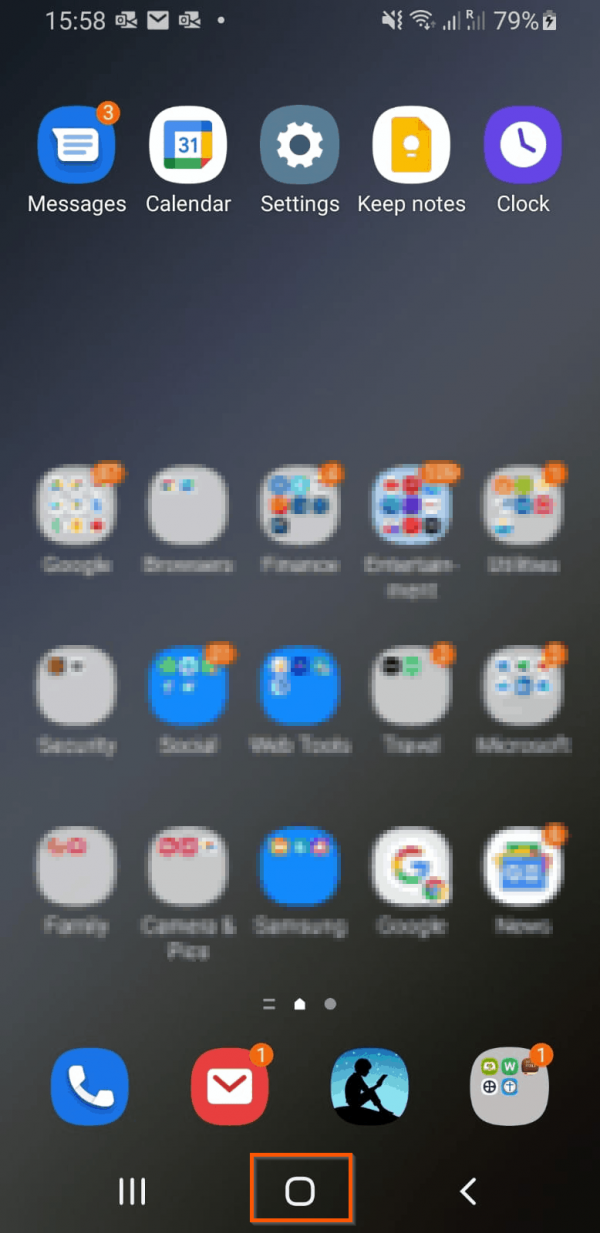This is a detailed screenshot of a smartphone's home screen, characterized by a predominantly black background. At the top, several apps are clearly visible, including Messages (with three unread messages), Calendar, Settings, Keep Notes, and Clock. Below these, a variety of apps are displayed, although not as clearly; these include Google, browsers, favorites, entertainments, Wi-Fi, security, sound, web task, TURL, Microsoft, family, Samsung, Facebook, Google, Facebook, an unknown app, pen, Google again, and an icon labeled "Jada".

At the bottom of the screen, there are easily recognizable icons for phone and messaging, with one unread message. The user also has an app icon featuring the silhouette of a boy reading a book against a light teal background, which stands out visually. Additionally, there's an app without a labeled name. The navigational interface includes three slashed marks, a home button, and a back button, completing the layout of the screen.